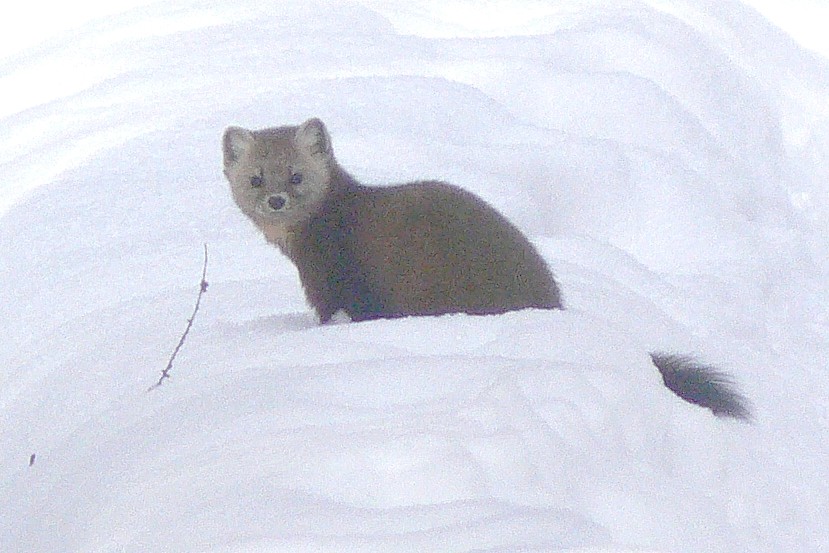In the center of the image, a small fox is staring directly at the camera. The fox's fur is primarily a reddish-brown color, with a lighter, off-white hue around its nose and inner ears. Its tail appears darker, almost black. Positioned to the left side of the fox is a single, long stem or twig emerging from deep snow that covers the ground entirely, without any other visible vegetation. There is a higher bank of snow behind the fox and a lower area in front, likely where the photographer is standing. The scene is set outdoors, in the middle of the day, under overcast skies, giving the image a palette of white, gray, light brown, dark brown, and black tones. The snow is so deep that the fox's legs are completely obscured, blending seamlessly into the wintry landscape.